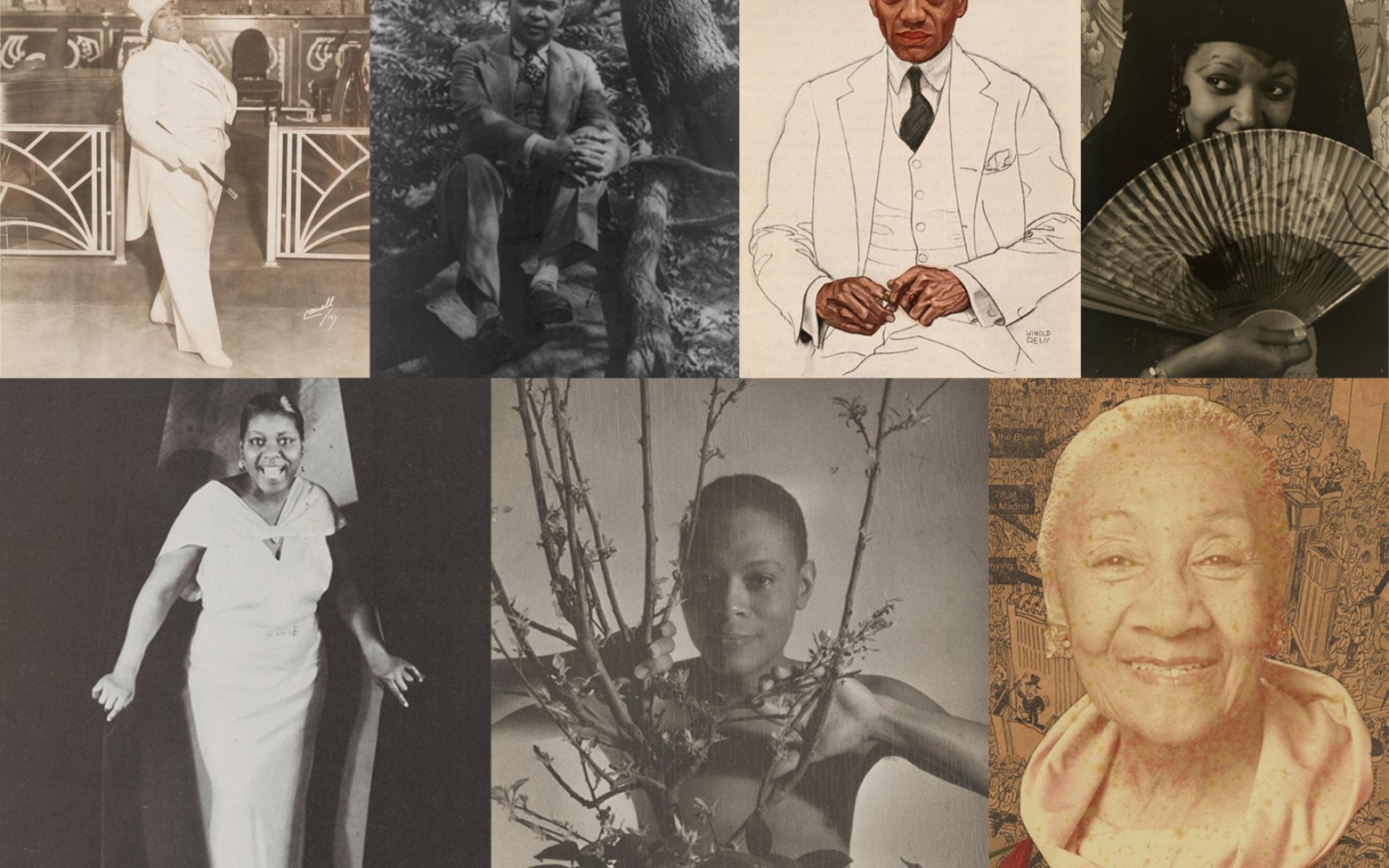The image is a collage of seven distinct photographs, each featuring African American individuals dressed in formal, elegant attire. In the top row, the first photograph on the left captures a black woman in an all-white suit and hat, standing against a white fence. Next, there is a black man dressed in a suit, seated amongst trees with his legs crossed and hands resting on his knees. The following image is a stylized black and white drawing of a black man, with only his hands and face colored in black. The final photograph in the top row depicts a black woman partially hiding her face behind a fan.

The bottom row starts with a photo of a black woman in a dress emerging from behind a curtain, her joyful expression clearly visible. The next image shows another black woman looking through tree branches, her hands gently holding the branches as she smiles. The last photograph in the collage features an older black woman, radiantly smiling, with a large, white fabric collar that frames her face, while the image itself has a sepia-toned hue. Together, these photographs create a rich tapestry celebrating the dignity and grace of black individuals, both young and old.